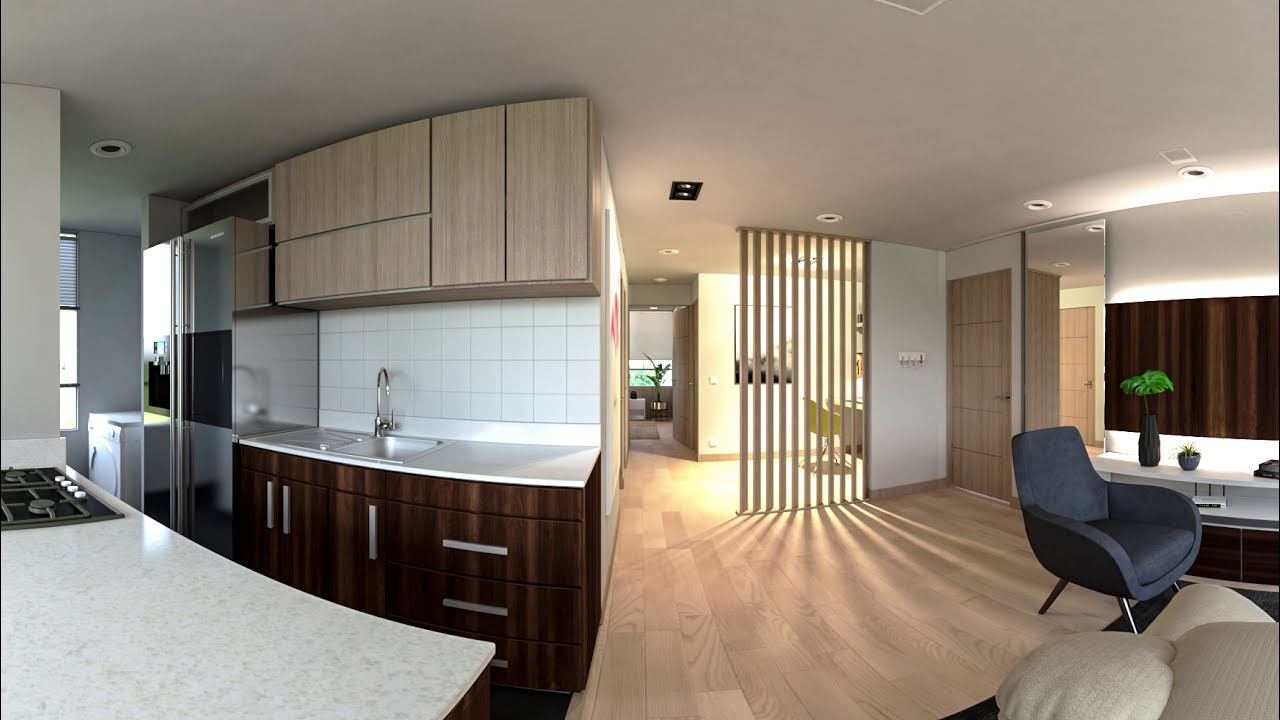This image depicts the interior of a multifunctional living space that likely serves as both a kitchen and an office area, captured with a fisheye lens that distorts the view slightly. The scene features a well-equipped kitchenette to the left with a white countertop housing gas burners and a stovetop. Above and below the kitchen sink are cabinets, and a large French door refrigerator is noticeable with a washing machine visible in the distant corner. A hallway extends from the kitchen area to other rooms, with light filtering in suggesting a slatted wall divider. To the right, the scene transitions into an office or living space, distinguished by a blue chair and a low shelf adorned with plants. The room also features a yellow chair near a mirror and a console table with additional plants, suggesting a cozy and well-decorated environment. The color palette includes neutral tones of tan, cream, white, brown, dark brown, beige, dark gray, black, and hints of silver, indicating a modern aesthetic. Light streaming through the windows implies it is daytime, confirming an inviting and airy atmosphere typical of an apartment, condo, or townhome.